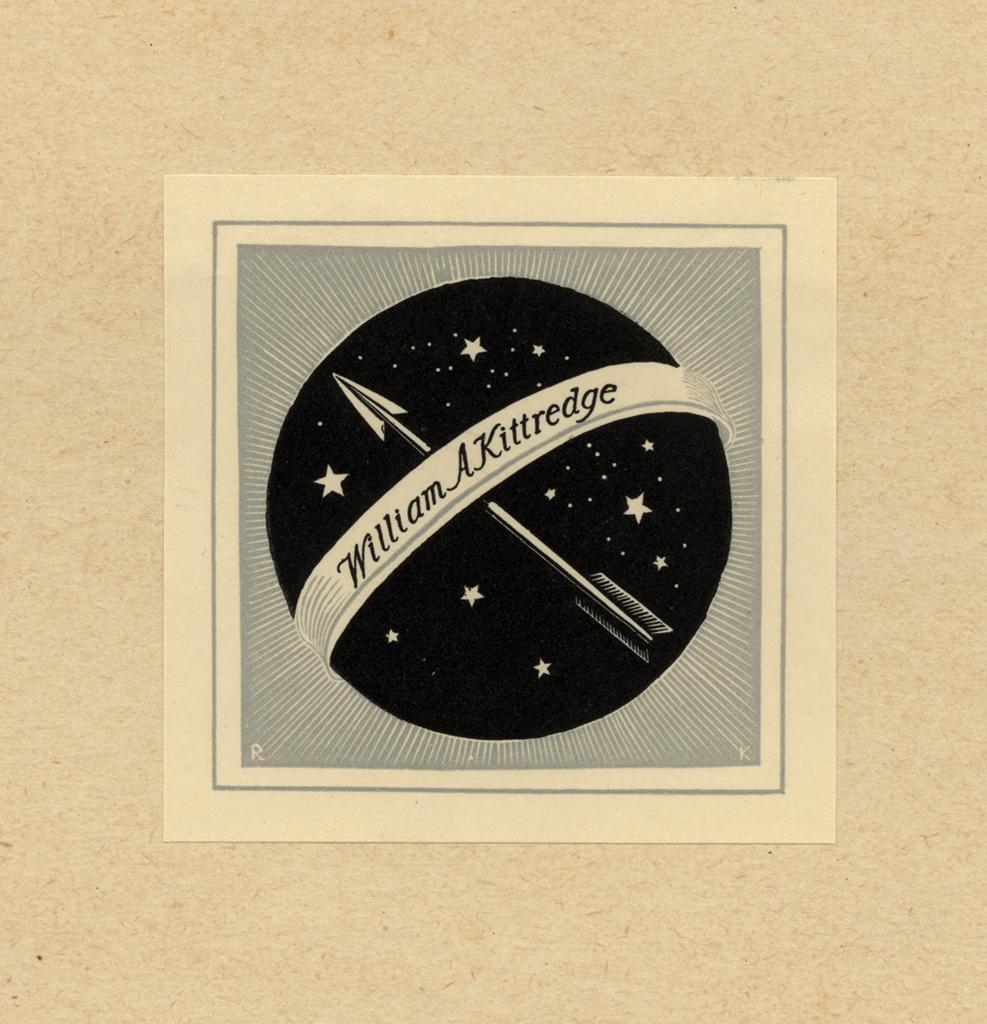The image is a detailed piece of artwork featuring an artist's signature, William A. Kittredge, prominently displayed on an off-white banner that wraps around a central black circle. Within this circle is a depiction of a night sky filled with both large, star-shaped stars and small dots, and a silver arrow pointing diagonally upward to the left. The circle is set against a lighter tan or cardboard-textured background with numerous thin, grey lines radiating outwards in various directions. The entire piece is bordered by a dark grey frame, and the larger tan border surrounding the entirety gives the impression of the artwork being affixed to a flat surface, likely a table. Additional details include the letters "R" and "K" situated at the bottom left and right, respectively.